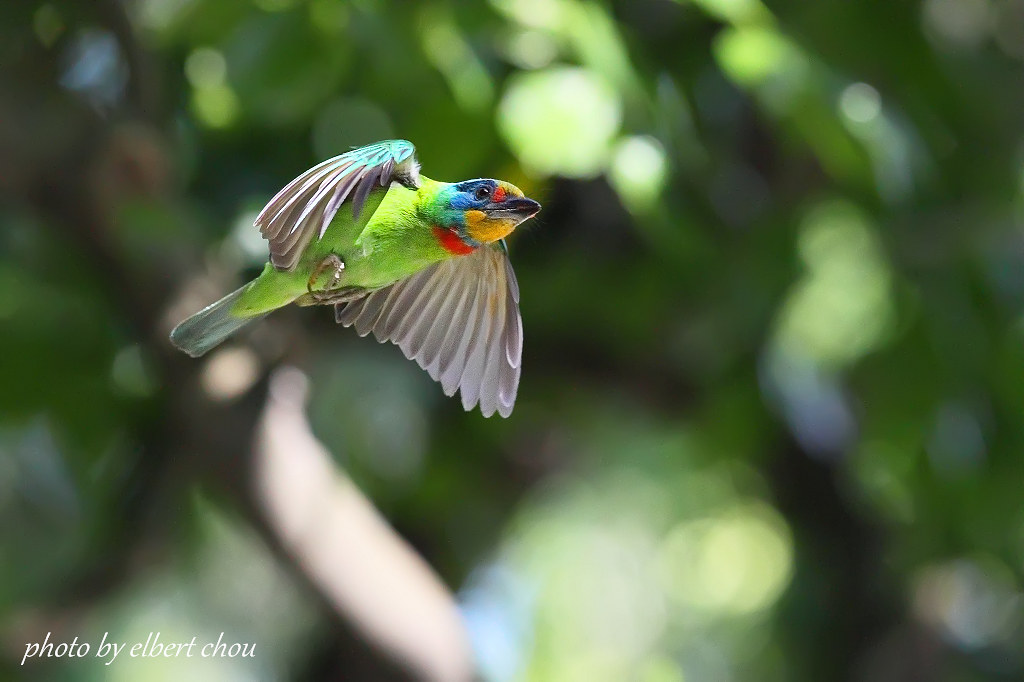This vivid, full-color photograph captures a Taiwan barbette mid-flight, set against a sunlit, blurry background of greenery and tree branches. The small-sized bird, roughly comparable to a sparrow, is slightly left of the image's center. It has a brilliant lime green body with striking multi-colored markings on its head: dark blue around the eyes, a yellow forehead, red patches near the beak and under the neck, and a touch of lighter blue and turquoise blending between the head and body. The wings are spread wide, showing white undersides and possibly blue tops, with its feet tucked underneath. Sunlight beautifully highlights the bird and the surrounding leaves. In the bottom left corner, white text reads, "photo by Albert Chou."